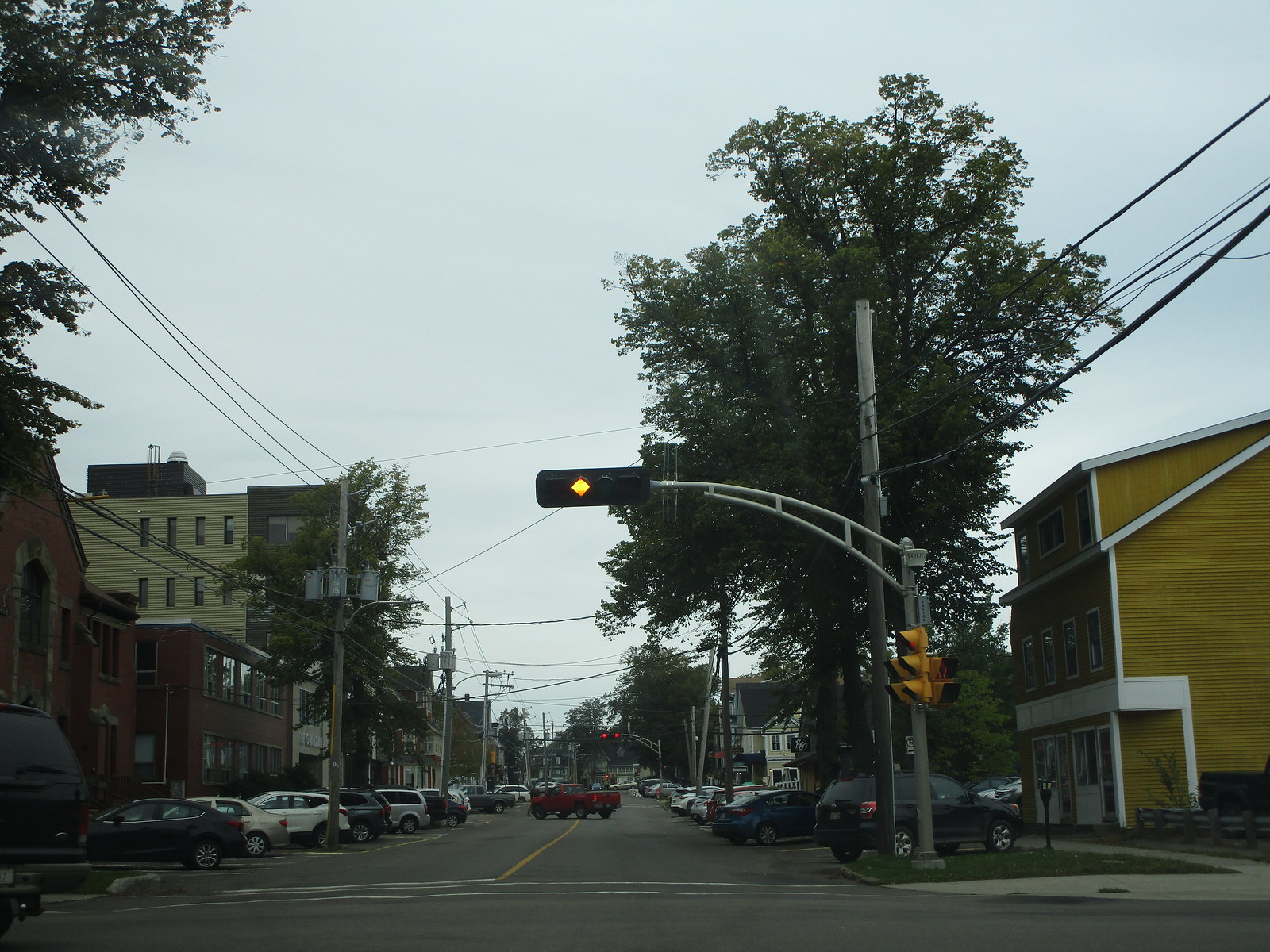A realistic photo taken from inside a car captures a typical street scene in a town. The vehicle appears to be approaching a stoplight, which is yellow, indicating the car is likely slowing down to stop. Unusually, the stoplight is horizontal, connected to a diagonal metal pole that also supports lights for the opposite direction. 

The street is lined with parked cars on both sides. On the left, a sequence of vehicles includes a black car, a gold car, a white car, a gray car, another white car, a black car, and a silver truck at the end. A red truck is in the middle of the road, making a turn. The right side of the road features a gray truck, a blue car, another white car, among other parked vehicles. Buildings flank the street: a yellow one on the right and a combination brick and yellow building on the left.